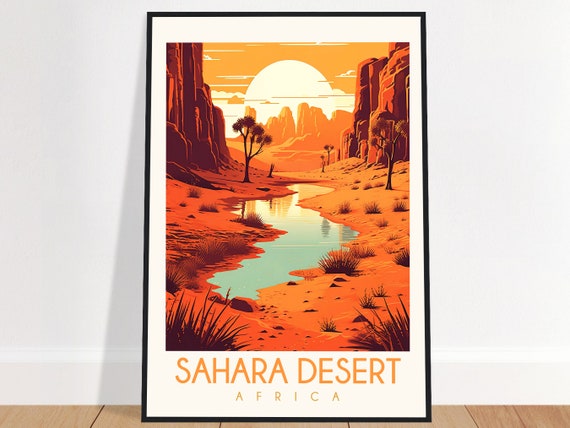In the image, a framed poster with a thin black border and a white mat is prominently displayed, leaning against a white wall with light brown hardwood floor beneath it. This striking poster, with an overall palette of oranges and browns, depicts a serene yet rugged desert landscape. Central to the illustration is a meandering creek, which starts as a bluish pool at the foreground and transitions to a golden hue toward the background. Flanking this creek are large rocky cliffs and spiky-leaved shrubs resembling Joshua trees at the bottom corners. The sky is an intense orange, set against a bright yellow sun that dominates the scene. The bottom of the poster bears the inscription "Sahara Desert, Africa" with "Sahara Desert" in a larger font size and "Africa" in a smaller one. The background details include plain white molding at the base of the wall, accentuating the simplicity and focus on the vibrant desert poster.